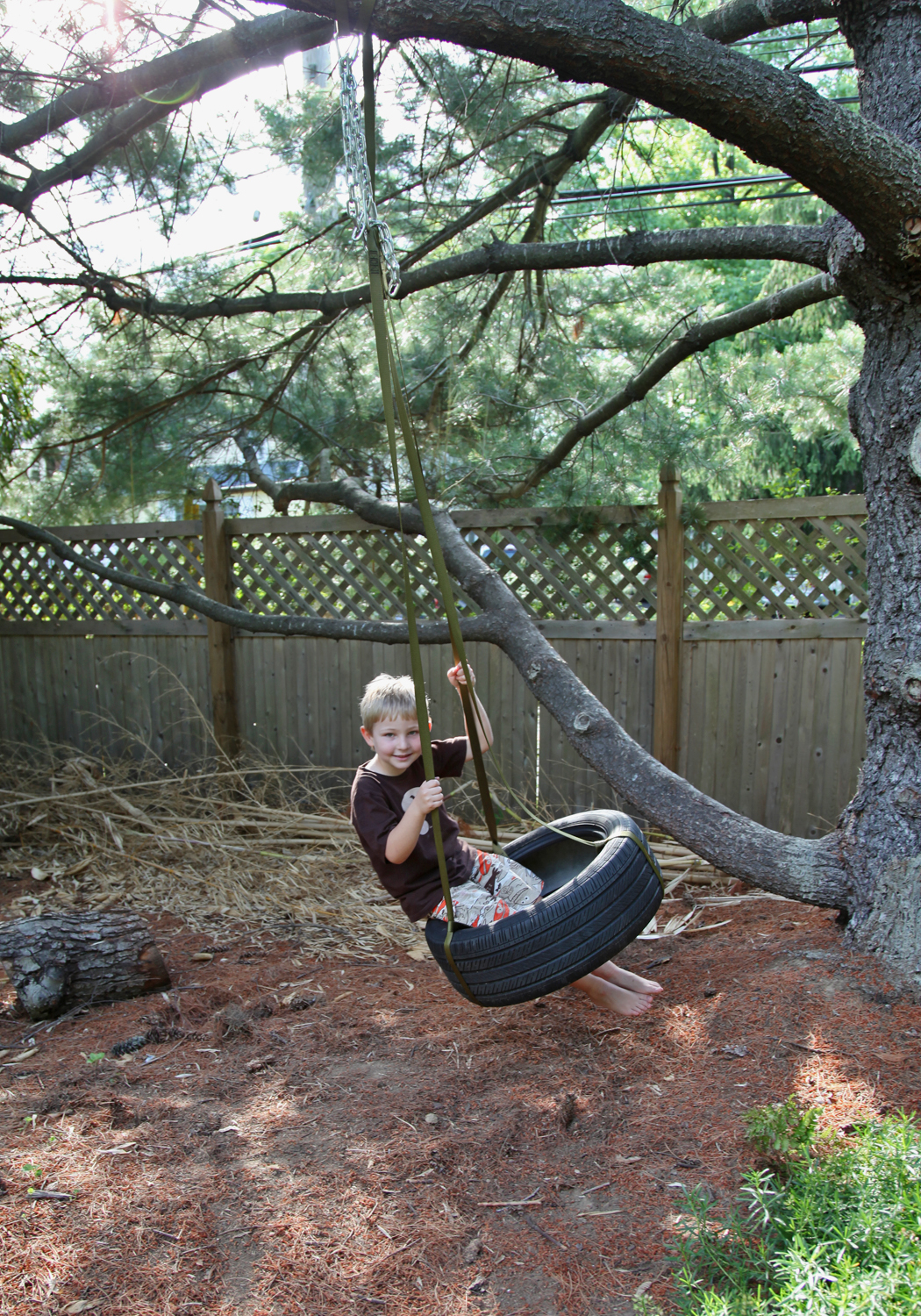In this photograph, a young boy with short blonde hair is joyfully sitting on a tire swing. He clings to the green ropes connected to short chains that suspend the tire from a sturdy tree branch. The boy, wearing a brown t-shirt and light shorts with an orange and brown pattern, is barefoot, adding to the carefree atmosphere. The scene captures the swing in motion, suggesting active play. Beneath the swing, the ground is a mix of dirt and grass, and to the right, an old tree with sprawling branches nearly touches the ground, possibly indicating it's partially buried. In the background, there's an old wooden fence, hinting this quaint, playful setting is likely a backyard.